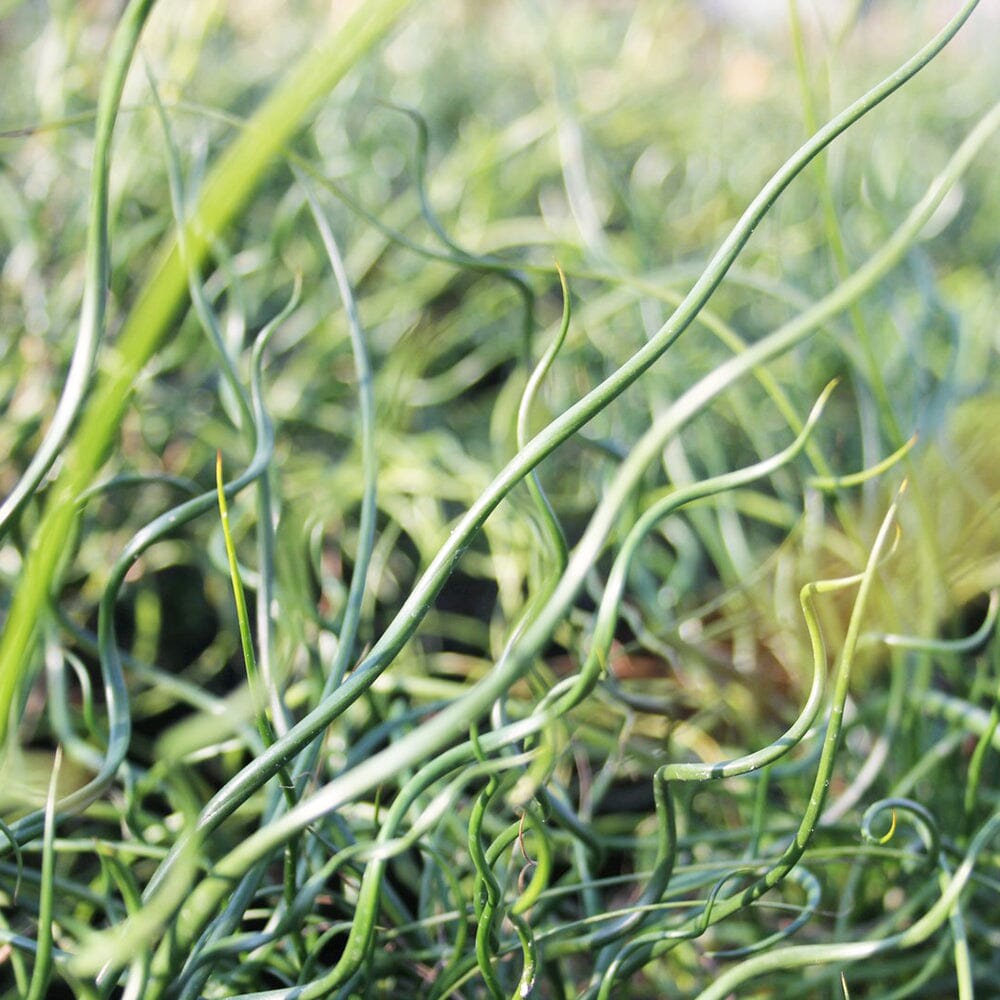The image captures an outdoor setting with bright natural lighting, suggesting it's taken during the day, and hints of what appears to be the sky at the top of the frame. The focus is mainly on the lower part of the image, which features an intricate and dense tangle of green strands, likely representing various types of grass or plants. These strands vary in shades of green, ranging from bright to darker greens, and are intertwined in a chaotic, twisting manner. Some strands have an appearance of cylindrical shapes, while others look flat, leading to speculation that they could either be plant stems or some sort of green cords. Prominently, one large strand extends from the bottom left corner diagonally to the top right, with sections of it curling and looping back. Several smaller strands also arc and twist amongst each other, with some maintaining a clearer focus in the lower right corner where a white-tipped strand stands out. The background appears blurry, filled with more indistinct green strands, enhancing the sense of a thick, tangled mass of plant life.